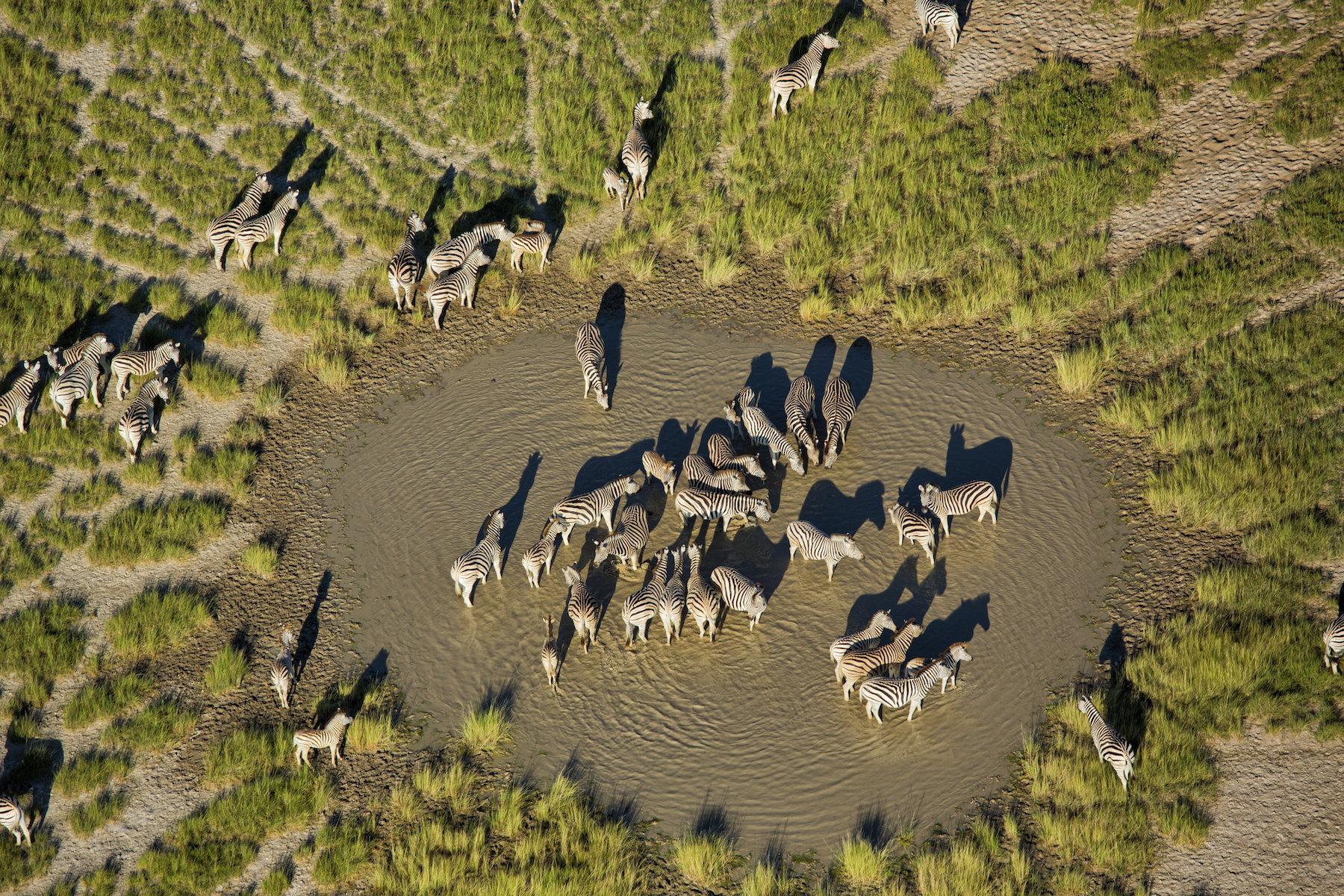An aerial view captures a serene scene in an African savanna, centered around a murky, circular pond. Numerous zebras stand in the shallow water, drinking and cooling off, while others roam the surrounding grassy terrain. Distinct dirt paths, created by the zebras' frequent journeys to the pond, are visible cutting through the grassland. In the bottom right corner of the image, there is a large, bare dirt area, and similar patches of light gray or light brown dirt are scattered in the top right, surrounded by sparse vegetation. Despite some blurriness, the image reveals a variety of zebras, including a few smaller ones that could be foals. Most zebras are calm and relaxed, though a few on the periphery appear vigilant, possibly standing guard. The overhead perspective emphasizes the zebras' natural behavior and the landscape's contrasting textures of grass, dirt, and water.